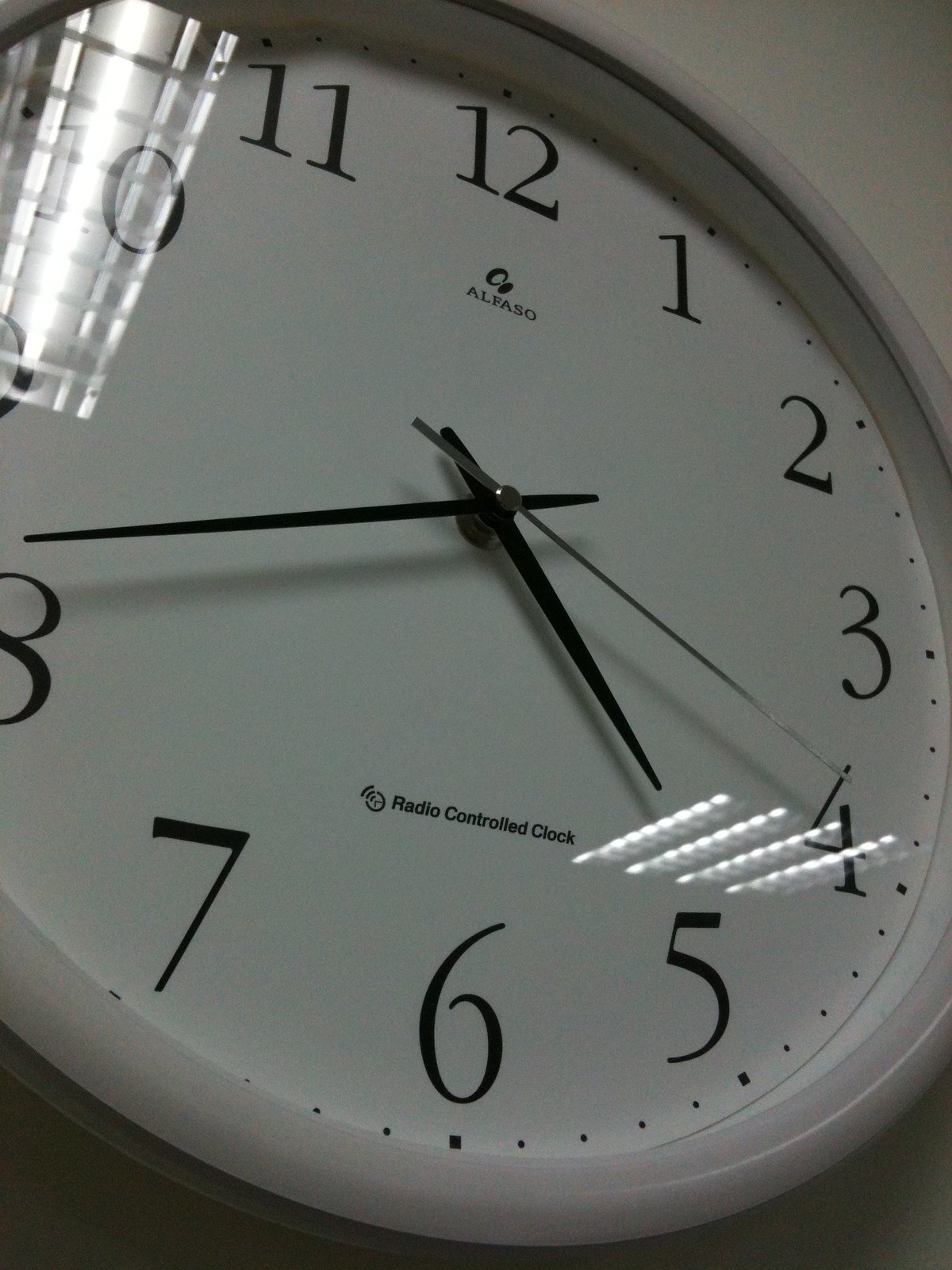This is a detailed, angled view looking upwards at a large, white wall clock. The clock face prominently features black numbers encircling its perimeter. The hour and minute hands are black and slender, contrasting with the silver seconds hand. Reflections play a significant role in this image; a large fluorescent light fixture is reflected at the top left of the clock face. Additionally, between the numbers four and five, there are four distinct white lines reflecting more fluorescent light fixtures. Centered at the bottom of the clock face, just above the number six, the text reads "Radio-Controlled Clock." Below the number twelve, the clock maker's name, "Alfazo," is clearly visible.